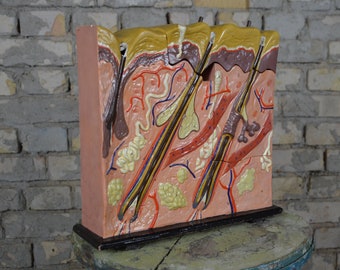The image depicts a detailed 3D model of skin layers, vividly illustrated and positioned on a marble table. The backdrop features a pattern of stone bricks in varying shades of gray, light gray, yellow, and pink, lending a rustic feel that could suggest an indoor setting or outdoor patio. The skin model itself is prominently square-shaped, resting atop a black stand. It showcases multiple layers: a topmost yellow layer transitioning to a darker brown, then a lighter brown layer, beneath which are shades of pink and purple. Dark brown hair shafts and red capillaries intersperse the model, accentuating key features. Yellowish pockets, likely representing fat or oil glands, are also dispersed throughout the structure, providing an intricate and educational representation of the skin's composition.